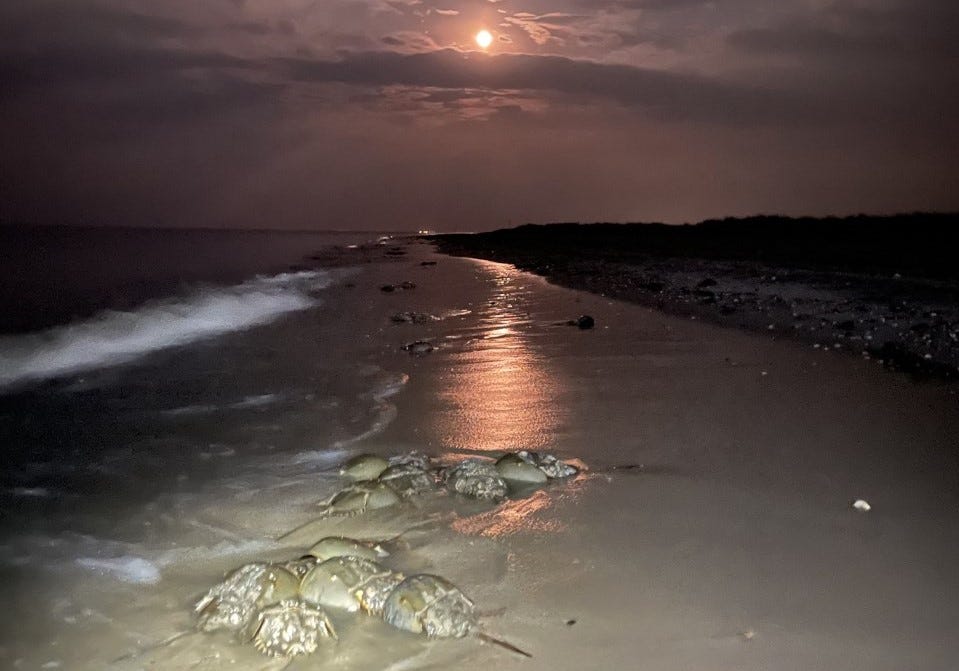The image captures a stunning sunset beach scene, where the sky is painted in hues of purplish-red, casting a serene glow across the entire landscape. At the very center top, the setting sun peeks out from above a cloud that resembles a hill, illuminating a strip of the beach with a faint pinkish-orange light. The horizon line sits in the top third of the photo, while the shorelines run towards the viewer.

On the far left, the ocean waves, tinged with gray and frothy white, are seen ebbing and flowing. In contrast, the right side of the image becomes dark and indistinct, suggesting either gravel marking the end of the beach or a rocky outcropping.

Dominating the foreground are numerous small crustaceans, possibly horseshoe crabs, clustered together on the damp, grayish sand. These rough-shelled creatures, resembling half of a helmet with sharp tails, appear trapped, awaiting the next wave to rescue them. Their beige coloring blends seamlessly with the sandy beach. Atop their shells, one can notice formations of microbiota, adding intricate details to the scene.

Above it all, the dusky lilac clouds create a dramatic backdrop against the faintly visible, pinkish-orange sunset, completing this picturesque and detailed beach scene.